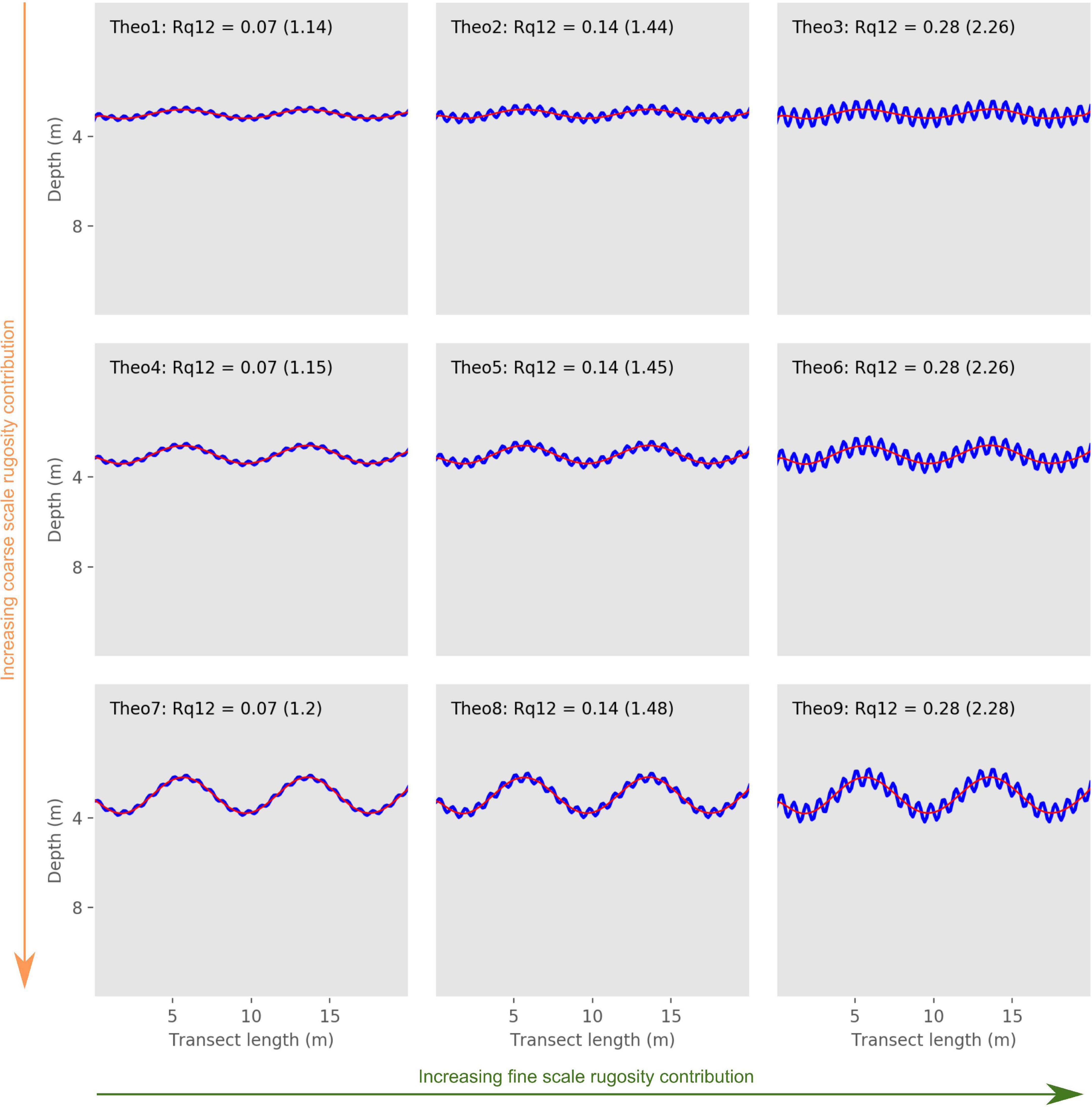The image consists of a grid with nine gray boxes, each containing a squiggly purple line that flows just above the center. As you move from left to right, the squiggly lines gradually increase in size and height. In the top left corner of each gray box, there is black text reading "TA201: RQ12 = 0.07 (1.14)," with a unique value for each box. Above the grid, a green horizontal line with an arrow points right, labeled "increasing fine scale rugosity contribution." Below the grid, the horizontal axis is marked "transect length" with values at 5, 10, and 15. On the left side of the image, an orange vertical arrow points downwards, labeled "increasing coarse scale rugosity contribution," followed by black text indicating depth values of 4 and 8 next to the respective rows. The chart provides a detailed visual representation of data with an emphasis on changes in rugosity and depth.